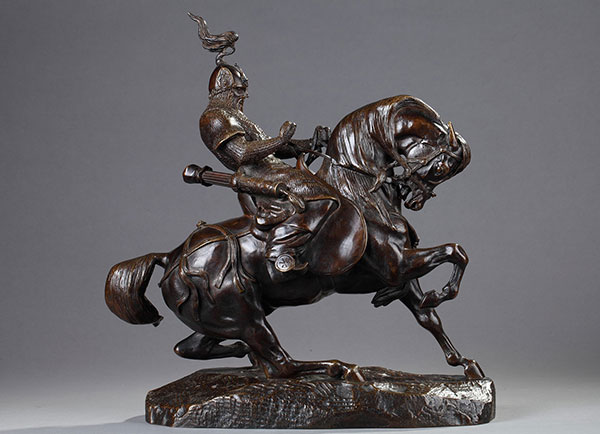The image depicts a bronze-brown colored statue, seemingly crafted from either hard plastic, bronze, wood, or a combination thereof, against a plain gray background. The statue showcases a knight, wearing detailed armor and a helmet adorned with a bird-shaped ornament. The knight is mounted on a dynamically posed horse, which is rearing up with its right front leg lifted and head bowed. The knight, gripping a sword at his side, appears steadfast and poised for action. The statue is set on a silver base about an inch tall and casts discernible shadows, indicating it rests on a white surface—potentially giving the impression of a product display for sale.